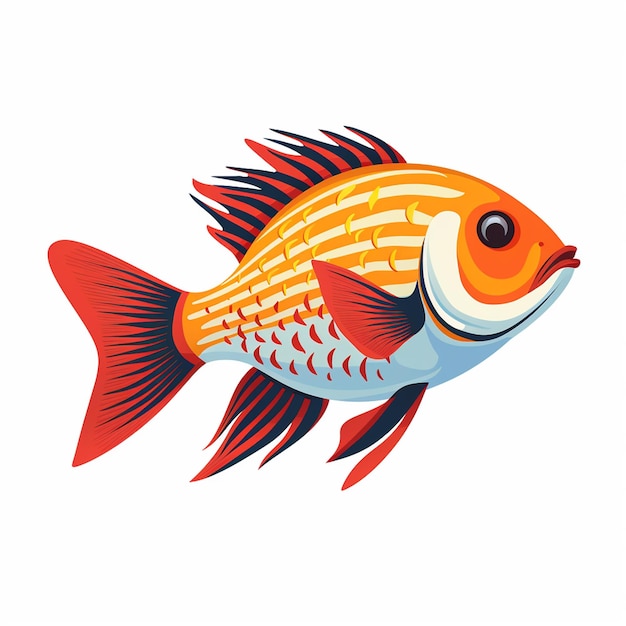This detailed square-shaped artwork, measuring approximately four inches by four inches, showcases a vividly drawn fish against a pale, off-white backdrop. The fish, resembling a goldfish but distinct in its own right, faces towards the right with a narrow, pointed nose that broadens through the middle before tapering into a V-shaped tail. The body of the fish is oval-shaped, almost flounder-like, adorned with horizontal orange and white stripes. Tiny red, boomerang-shaped markings and yellow dashes accentuate its vibrant body.

The fish features various fins, including spiky dorsal fins, wavy bottom fins near the tail, and a single side fin. These fins are predominantly dark orange or red with black stripes, and some contain dark blue lines. The fish's lips are a notable dark red, forming a distinct frown. Its eye is complex, with a black pupil encircled by white, and an outer black ring providing additional contrast.

White dominates the fish's underbelly, extending to the cheeks and the area beneath the chin, blending into the orange and dark orange shades around the eye and gills. The artwork's simplicity in the background emphasizes the detailed, colorful depiction of the fish, making it the centerpiece of the piece.